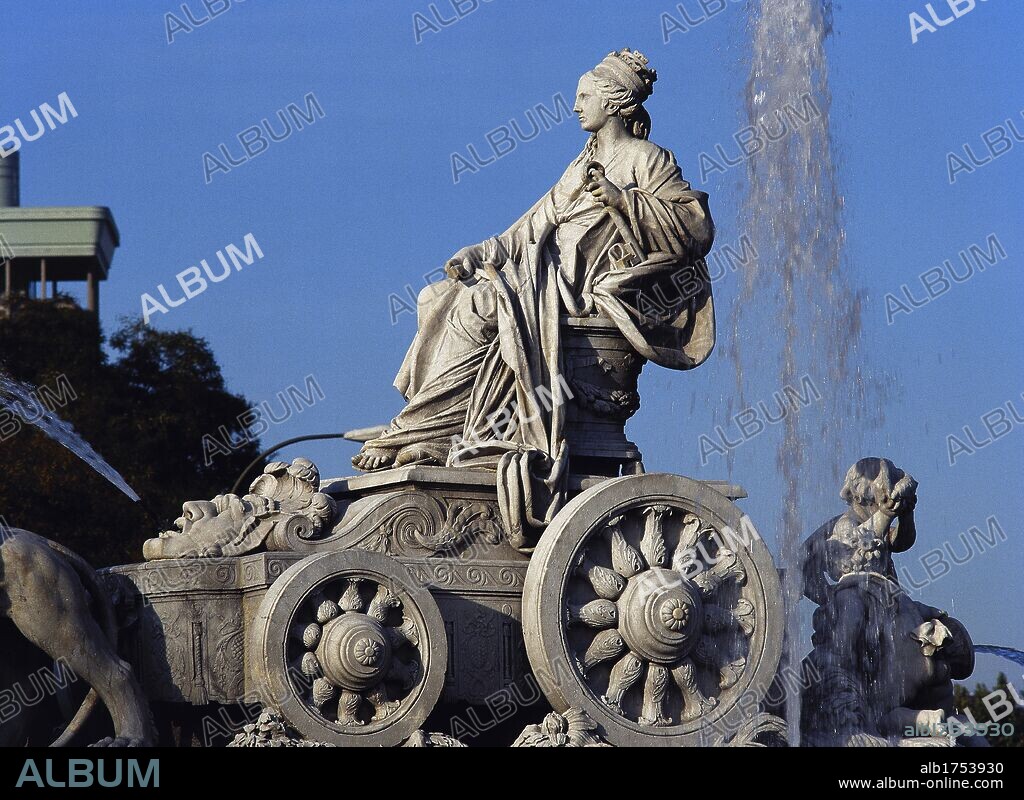The image portrays a detailed statue set against a bright blue sky, with the word "album" watermarked repeatedly across it and "albumonline.com" present in the bottom right corner, indicating ownership. The stone statue, reminiscent of European art, features a stoic woman with her hair up, draped in voluminous robes that expose her toes. She sits on an ornate chair placed atop a decorative wagon, which has a larger back wheel and a smaller front wheel. The wagon's spokes are intricately designed. A smaller statue, likely a child, is positioned behind the woman, near where water is seen flowing downwards, suggesting the structure functions as part of a fountain. Additionally, water is actively spraying mid-air on the right side of the image, reinforcing the fountain-like setting. The statue's positioning and these elaborate details create a captivating scene of historical and artistic significance.